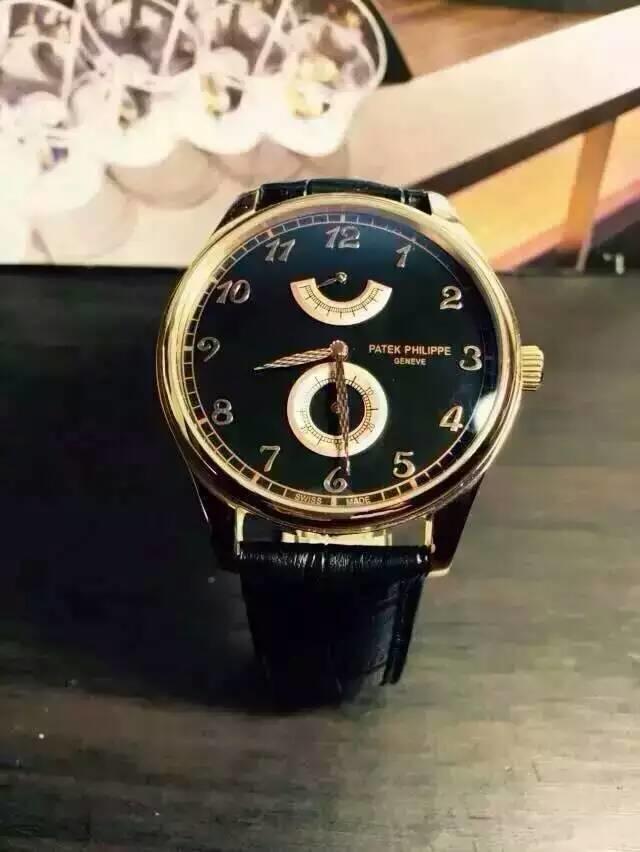The image showcases an elegant watch placed on a sleek black table. The timepiece features a sophisticated black leather wristband, enhancing its luxurious appeal. Its watch face is bordered in gold, including the crown, the small knob used for time adjustments. The numerals on the dial are also gold, contrasting beautifully with the deep black background of the watch face. The time on the watch is set to a few minutes before 8:30. Inscribed on the face, below the center, are the words "Swiss Made" and "Patek Philippe Genève," emphasizing the watch's prestigious heritage. Additionally, there is a date dial centrally positioned, and a distinctive half-moon shaped indicator located beneath the 12 o'clock mark, complete with a small pointer. In the background, a white shelf or display case is partially visible, adding to the refined context of the scene.